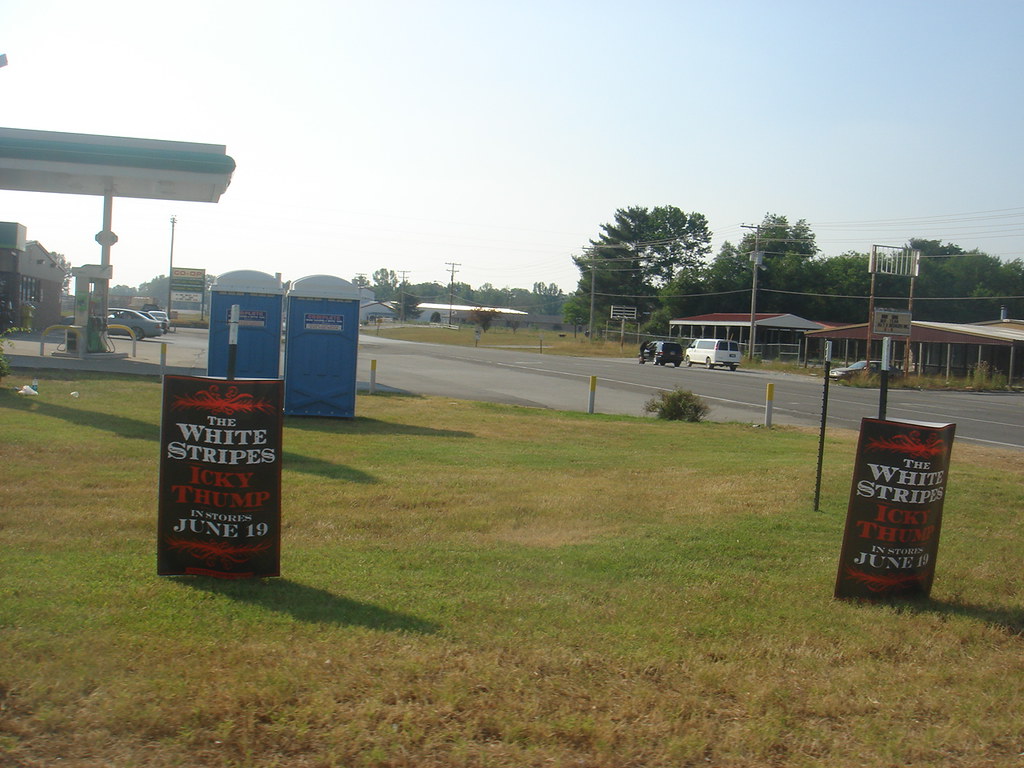The photograph, taken outdoors on a hazy, late afternoon, showcases a horizontally aligned landscape scene. The image is centered on a road that stretches from the upper left to the bottom right side. A grassy area with patches of green and brown sits to the left of the road. This area features two blue porta-potties and two metal rods holding black rectangular signs with red designs and white lettering that read "The White Stripes Icky Thump in stores June 19th." In the distance on this grassy area, there is a gas station, identifiable by its awning and petrol pumps. On the far side of the road, two single-story abandoned buildings with shallow pitched roofs stand side by side, with a white van and a black minivan parked alongside them. Timber posts with overhead power cables are visible along the road, and trees can be seen behind the buildings, contributing to the quaint yet desolate atmosphere of the scene.